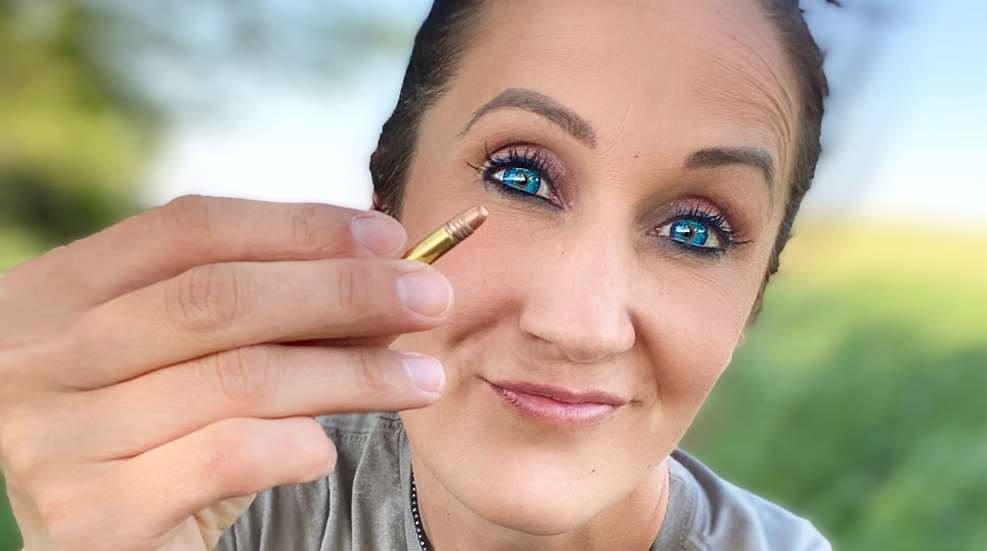The image is a highly detailed close-up of a smiling woman with strikingly bright blue eyes that appear almost unnatural in color. Her eyes are accentuated with heavy mascara, making her eyelashes look dense and slightly clumped together. She has sparse, painted-on eyebrows and her lips are adorned with a subtle, pinkish nude balm. The woman has brown hair, though the top of her forehead is cut off, and she is wearing a grey shirt. She is holding a slim, golden bullet between her index finger and thumb, presenting it towards the camera with an expression that seems to say, "Look at this." The background is blurry but suggests she is outdoors, with hints of a blue sky, green trees, and grass.